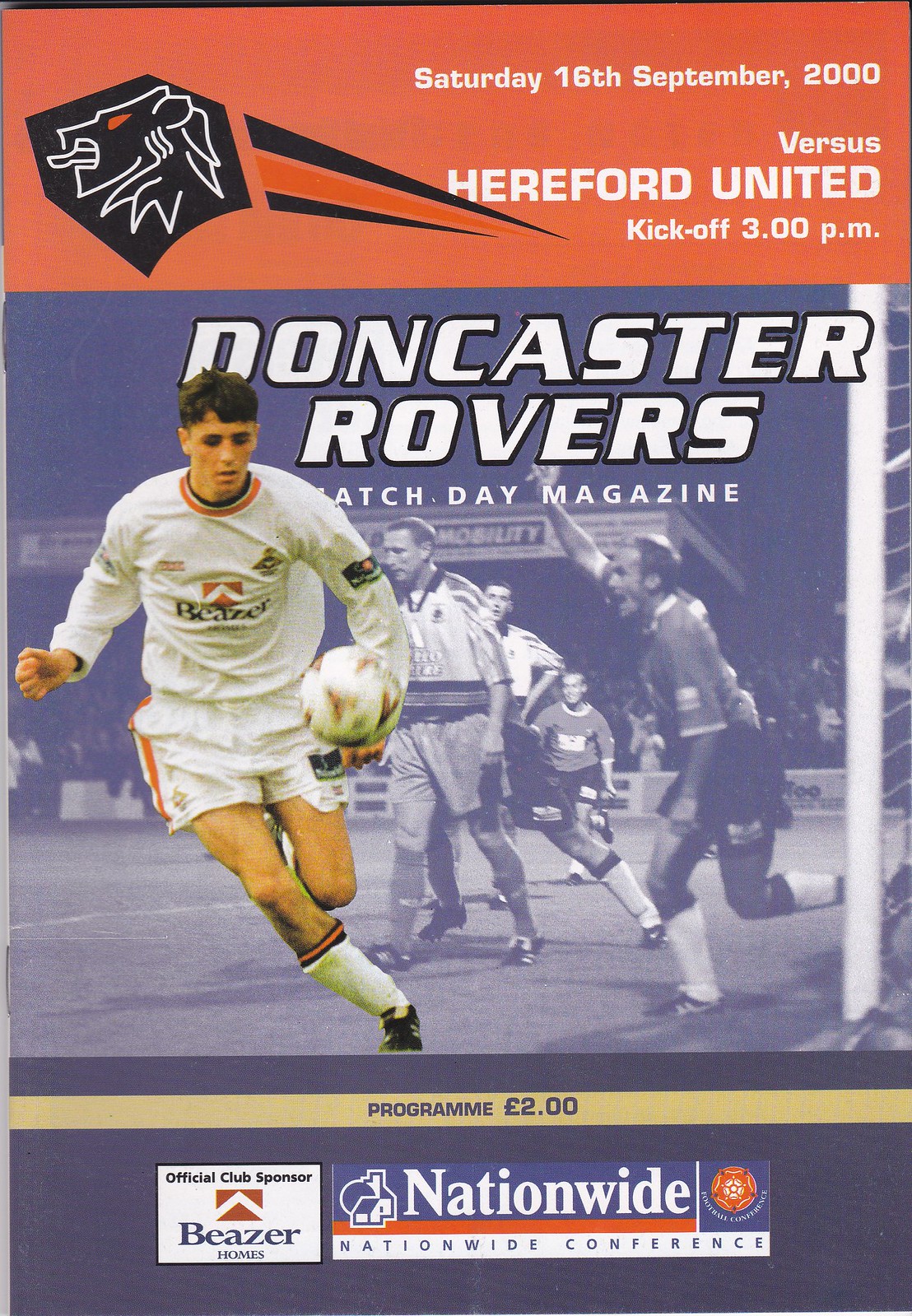**Magazine Cover Description:**

This magazine cover, primarily dark blue with accents of tan, orange, white, black, and gray, showcases a Doncaster Rovers matchday program from Saturday, 16th September 2000, for a game against Hereford United with a kickoff time of 3:00 pm. At the top-left, a prominent lion face logo sits on a red strip, next to the event details. Central to the cover is a vivid, color photograph of a football player in action, surrounded by other players against a backdrop of the playing field. Above this image, the title "Doncaster Rovers Matchday Magazine" is clearly displayed. The bottom of the cover features the program price, marked as £2.00, along with two sponsor logos: Beezer Homes, the official club sponsor, and Nationwide Conference, highlighted by an orange circle. The background of the main image contrasts richly as black and white, emphasizing the dynamic, colorful scene of the football player.